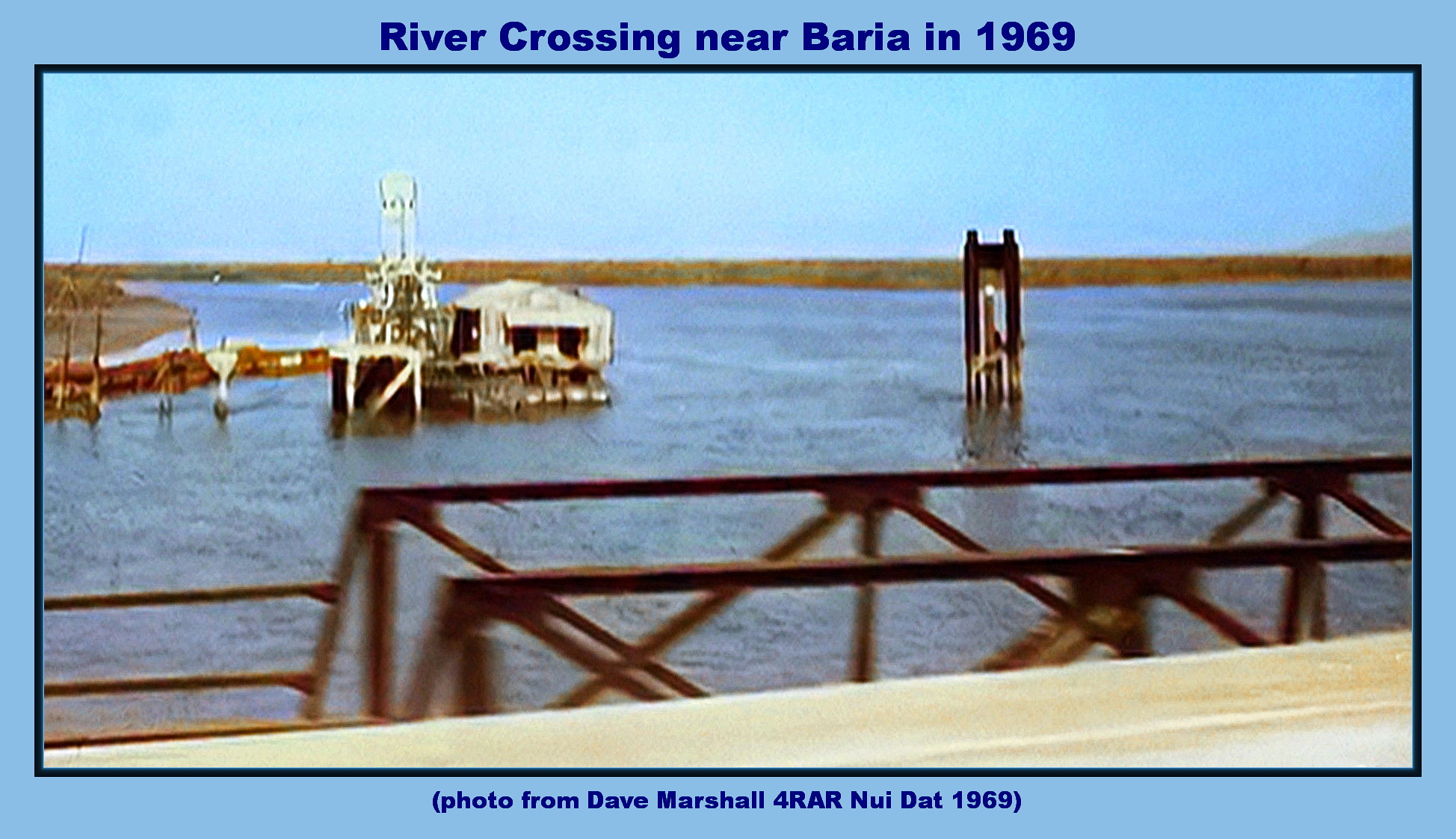This image, resembling an old postcard from 1969, captures a serene river crossing near Baria, Vietnam. Dominated by an expanse of clear blue skies and distant grassy landscapes, the scene is anchored by a waterway, possibly a river or lake. Central to the image is a white structure, which appears to be a small house or dock. Adjacent to it, on the left, a pump-like device can be seen, suggesting a use for oil or another utility. To the right of the house is a bridge or railing extending out over the water, hinting at a damaged or incomplete crossing. The photograph's setting casts a peaceful yet nostalgic aura, framed by a black border. Complementing the visual, blue lettering at the top reads "River Crossing near Baria in 1969," while the bottom showcases the inscription, "Photo from Dave Marshall for RAR Nui Dat, 1969." This detailed caption offers an evocative glimpse into the historical and geographical context of the scene captured by Dave Marshall.